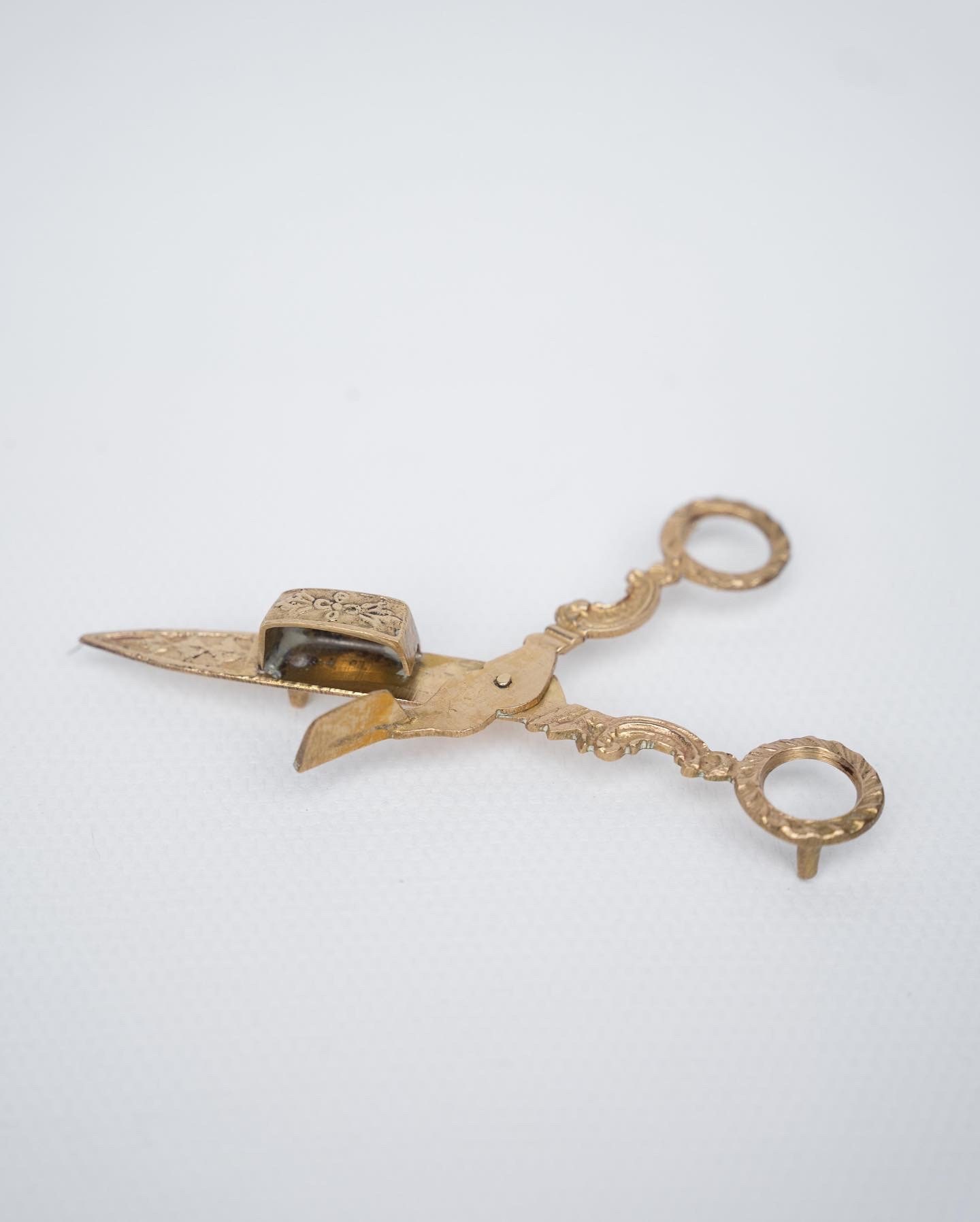This intricate photograph showcases a pair of vintage, gold-trimmed scissors resting on a white background. The scissors, ornate and possibly from a bygone era, are distinguished by their unique design features. One blade appears conventional, while the other is significantly shorter, suggesting it may be optimized for specialized tasks. The handles are elaborately decorated and wavy, showing floral filigree patterns, lending both functionality and artistic flair. Noteworthy is the peculiar set of small legs allowing the scissors to stand upright on any surface. The overall impression is one of an exquisitely crafted tool, combining functionality with aesthetic detail.